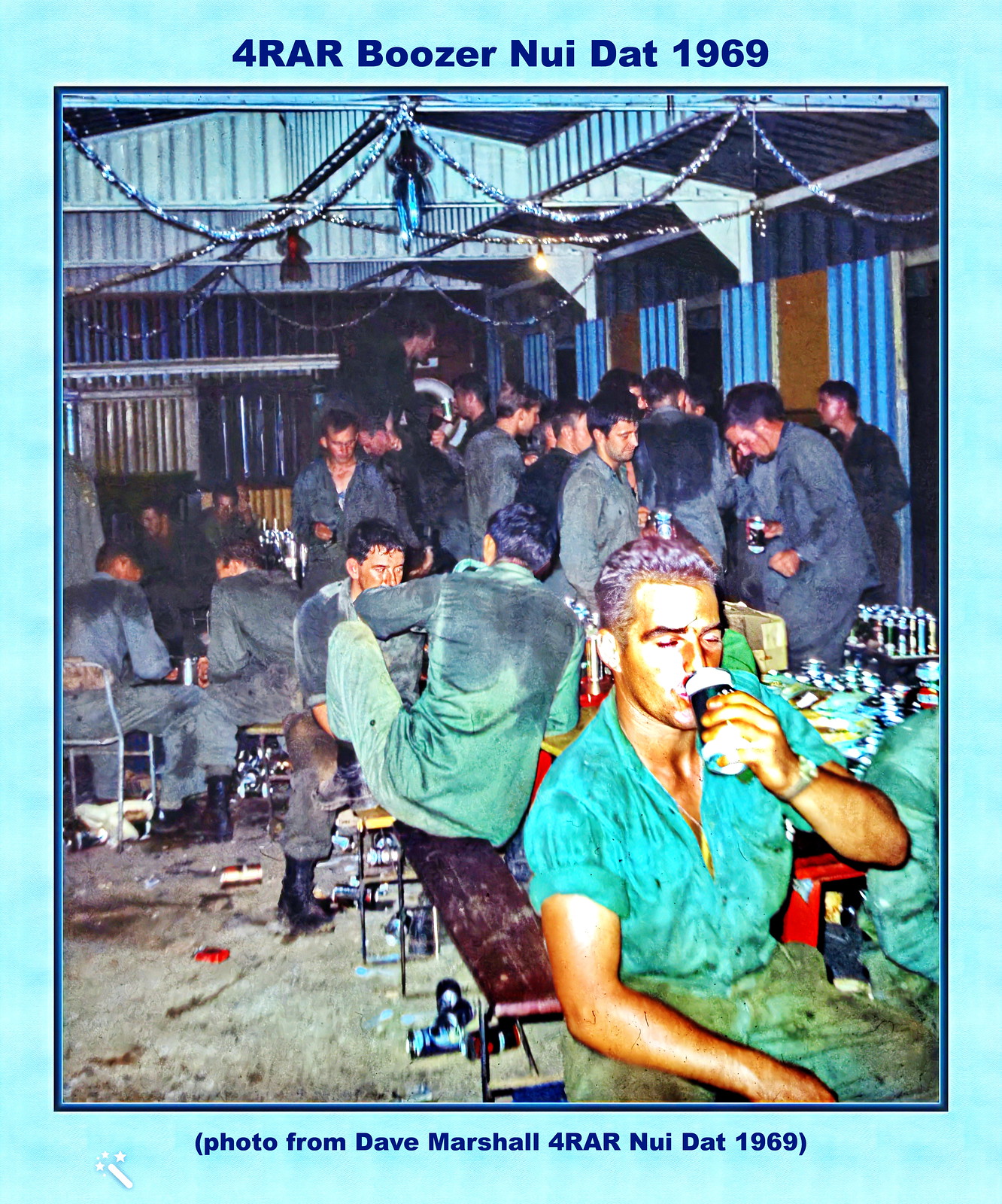The image features a colorized or color-tinted photograph inset within a light blue border, framed by dark blue text at the top and bottom. The top headline reads "For 4 RAR Boozer Nui Dat 1969," and the caption below notes "(Photo from Dave Marshall, For 4 RAR Nui Dat 1969)." The scene centers on a group of men, likely soldiers, gathered inside a somewhat dingy army facility in Vietnam. Most of them are seated at picnic tables, engaging in drinking and merriment, perhaps celebrating an event. The man in the bottom right corner, who is the most prominent, is wearing an aqua shirt and beige pants while holding a beer to his lips. The background includes corrugated blue and brown walls with matching panels overhead, adorned with silver tinsel streamers. The setting, colors, and clothing—ranging from light blue, dark blue, and green to tan and red—suggest a lively yet rugged environment. The overall style blends vintage photography with graphic elements, highlighting the communal and celebratory atmosphere amidst the harsh conditions.